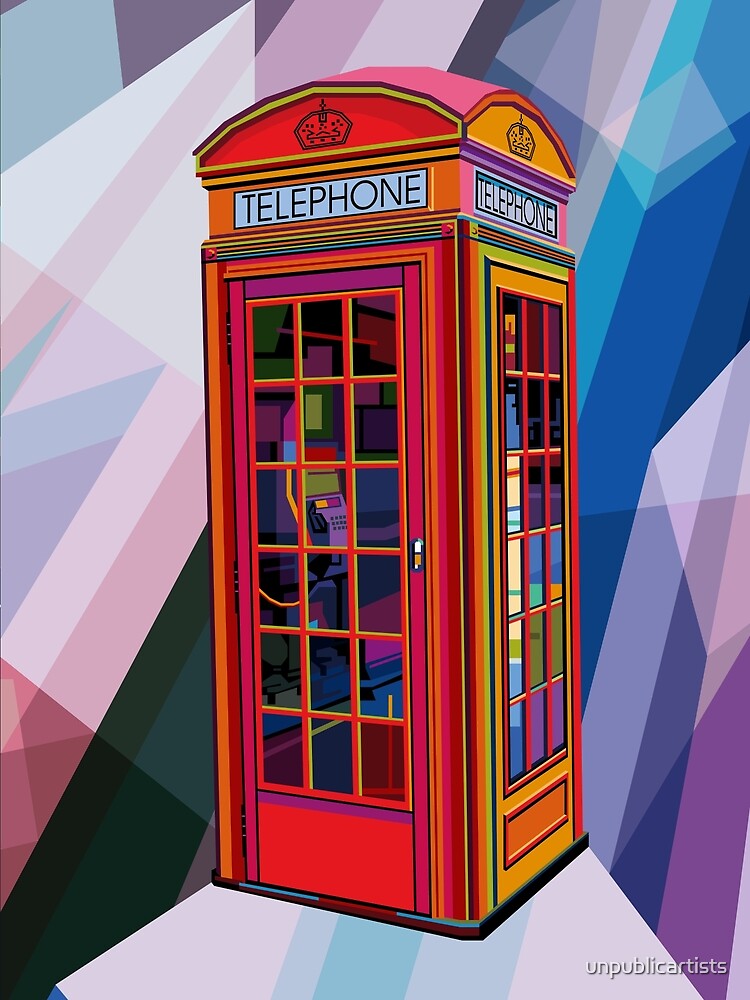The image is a vibrant and detailed digital drawing, presented in portrait mode, featuring a traditional English telephone booth that exudes a retro charm with modern artistic flair. This red telephone booth, reminiscent of the TARDIS from Doctor Who, is adorned with a British crown on top and bears the word "TELEPHONE" in white rectangles above the door and a side window. The multi-dimensional booth is colored in rich hues of red, orange, dark purple, and hints of green and blue, showcasing its many glass panes through which a purple telephone is visible inside.

The intricate background is an explosion of neon colors and geometric shapes, resembling crystals in shades of light pink, light blue, dark blue, and dark green, adding a dynamic and ultramodern context to the scene. Additionally, the artist's signature "UNPUBLICARTISTS" is discreetly placed in the bottom right-hand corner, marking the creative origin of this striking artwork.